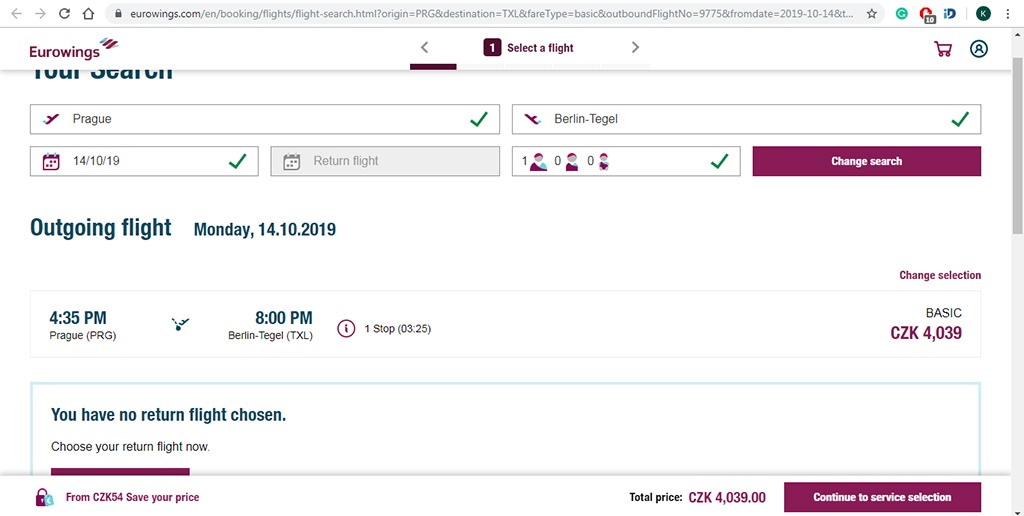This screenshot captures a desktop or laptop browser window open to an online flight booking interface for Eurowings. At the top of the browser, familiar navigation icons can be seen: a left-pointing arrow, a right-pointing arrow, a circular arrow for refreshing the page, and a house icon. The address bar displays the Eurowings website address, flanked by various icons on its right end.

Centrally positioned at the top of the page, the text "1. Select a flight" indicates the current step in the booking process. Below this heading, partially cut off yet readable, is a section for inputting search criteria. It shows a departure from Prague, highlighted with a checkmark, and a destination of Berlin Tegel, also checked.

On the left-hand side, information about the outgoing flight is detailed under the heading "Outgoing flight, Monday, 14-10-2019." Specific flight details are given: departure time from Prague at 4:35 p.m. and arrival time at Berlin Tegel at 8 p.m. On the right side of this line, the fare type is listed as "Basic C, ZK 4,039."

At the bottom of the screen, a message informs the user that no return flight has been chosen. This section also features a lock icon on the left side for security. On the right, a prompt states "Continue to service selection," guiding the user to the next step of the booking process.